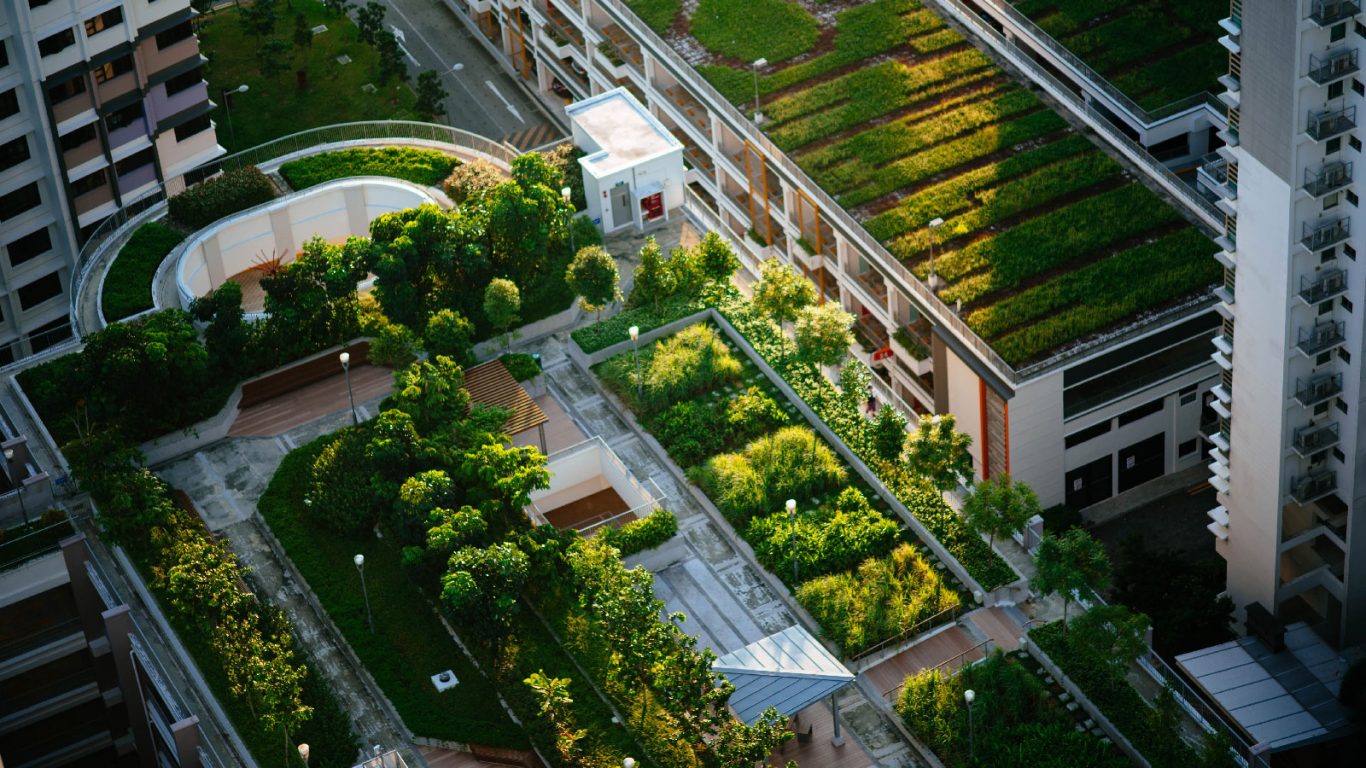The image is an aerial view of a densely packed urban area featuring several apartment buildings with innovative rooftop gardens. The buildings, approximately three stories high, lack ground-level green spaces, leading residents to create lush gardens on their roofs. One rooftop features horizontal rectangular plots cultivating garden vegetables like lettuce and carrots, with walkways lined with bark chunks. Another building across the street showcases more expansive rooftop greenery, resembling a mini park with trees, streetlights, picnic tables, and tree-lined sidewalks, where residents could walk dogs. This rooftop also hosts an orchard area with fruit trees and herbs such as rosemary, complete with white-painted wooden walkways. On the front-left building, there's a semi-circular section, and a generator is visible on the top right. Multiple lamp posts are installed around the gardens, enhancing the urban landscape with a touch of nature.